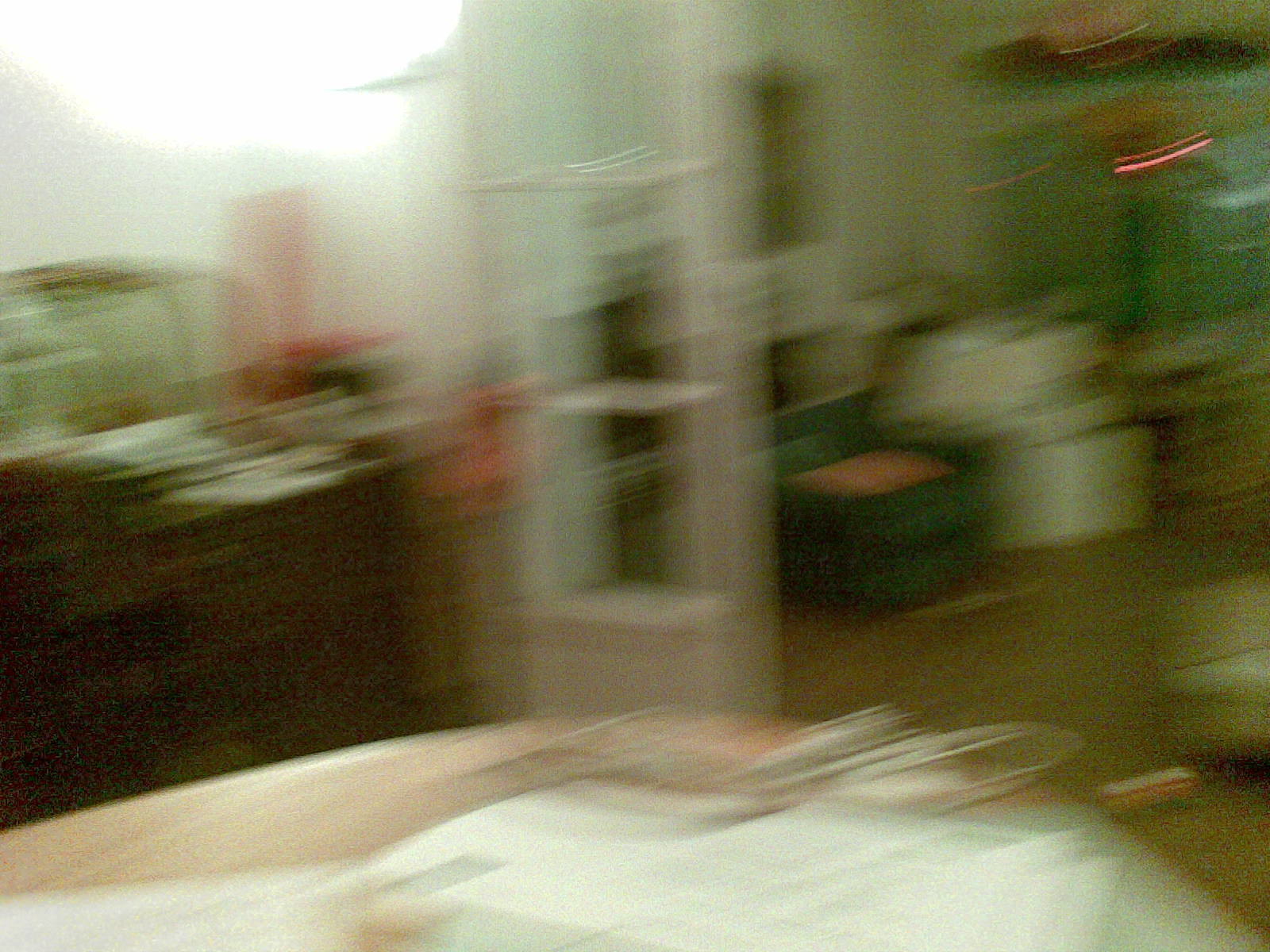The image presented is of extremely low quality and is notably grainy, making it challenging to discern specific details with clarity. At the bottom of the image, there is a significant white blur that could potentially represent a couch or a chair, surrounded by a whitish, translucent halo that makes identification difficult. Centered in the image is a white structure that appears to be either a ladder or a shelf, composed of three blurred, rectangular layers. To the left of this central object, there seems to be a dark wooden desk, though it is similarly obscured by the blurriness. Additionally, the overall photo quality is marred by white streaks. A light source is visible in the top left corner, contributing to the illumination of the scene. On the right side of the image, red streaks add to the colorful distortion, with possible glimpses of another chair or couch and perhaps a cabinet. The overwhelming graininess and lack of clarity render the precise details and arrangement of the objects in the image highly ambiguous.